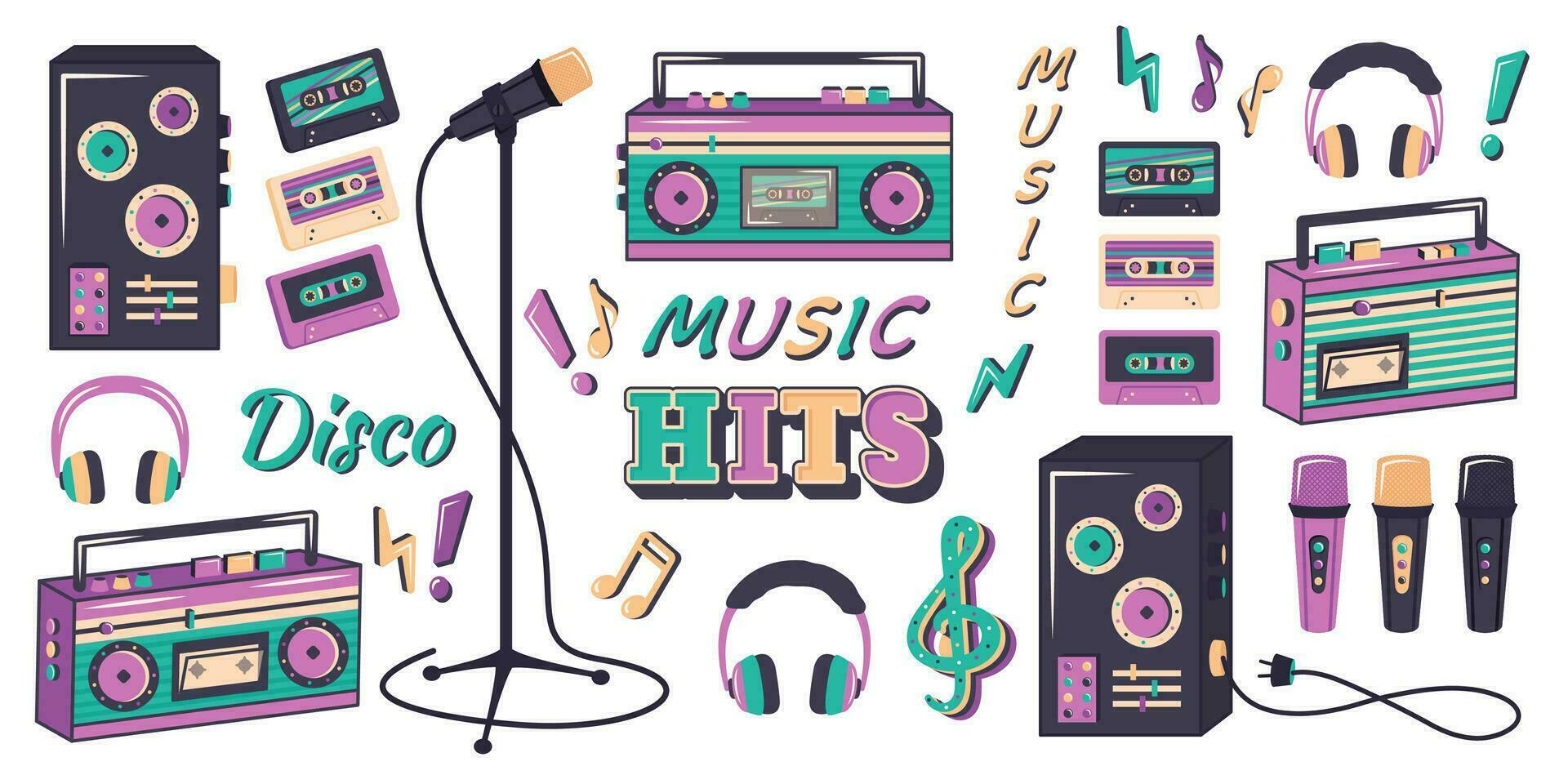The color image features a detailed assortment of hand-drawn, music-related objects arranged against a white background. The centerpiece is a boombox with purple speakers and a black border, while its body is a mix of purple and green, complete with control buttons and a handle. Among the array are three boomboxes in total, along with two speakers — one depicted with a power wire — and three sets of headphones. The scene also includes a black microphone atop a mic stand, three handheld microphones, and six cassette tapes.

The color palette prominently features shades of yellow, green (both light and dark), purple, and pink. Scattered text around the objects includes words like "Disco," "Music Hits," and "Music," with some words written vertically. Musical notations, such as notes and exclamation marks, enhance the thematic elements. A striking motif within the illustration is the repeated appearance of lightning bolts, underscoring the dynamic and energetic theme. The carefully placed elements, patterned with consistent hues of green and purple, create a vibrant, lively composition reflecting a nostalgic yet colorful celebration of music memorabilia.